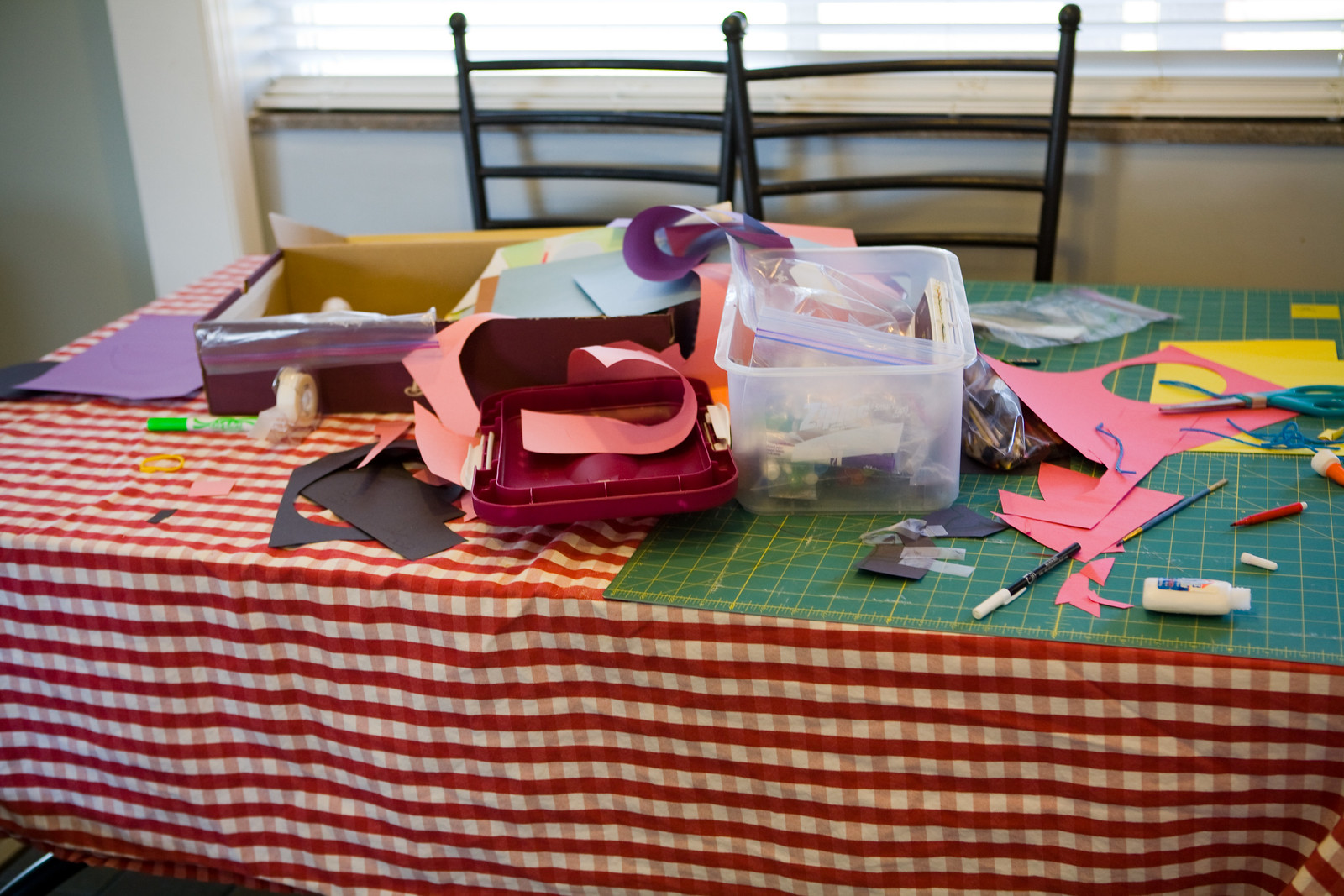A detailed and expansive array of arts and crafts supplies is meticulously arranged on a table indoors, likely situated in a cozy living room or kitchen space. The table is adorned with a red and white plaid tablecloth that resembles a picnic blanket, setting a charming and inviting scene. Atop the tablecloth is a green and yellow cutting mat, complete with ruler markings for precise measurements.

On the mat, assorted crafting tools and materials are spread out. A white marker with a black body and white cap lies next to a small bottle of Elmer's glue. Nearby, a blue and gold pencil is positioned alongside a red marker. An assortment of pink and yellow construction paper, some with large holes and others in smaller scraps, is scattered across the surface.

To the left, a clear plastic tub filled with additional arts and crafts supplies stands, partially obscured by the clutter. Its accompanying maroon-colored lid rests beside it, topped with yet another piece of pink construction paper. Behind this, a cardboard box is visible, containing various sheets of brown, blue, and orange construction paper along with other miscellaneous papers. Adjacent to the box is a piece of black construction paper, already cut into shapes, and a separate sheet of purple construction paper.

In the background, two metal chairs stand by, hinting at a space ready for creativity and collaboration. A window with open blinds lets in daylight, illuminating the entire scene with natural light. The surrounding wall is painted a serene, desaturated blue, completing the peaceful yet industrious atmosphere of this crafting haven.